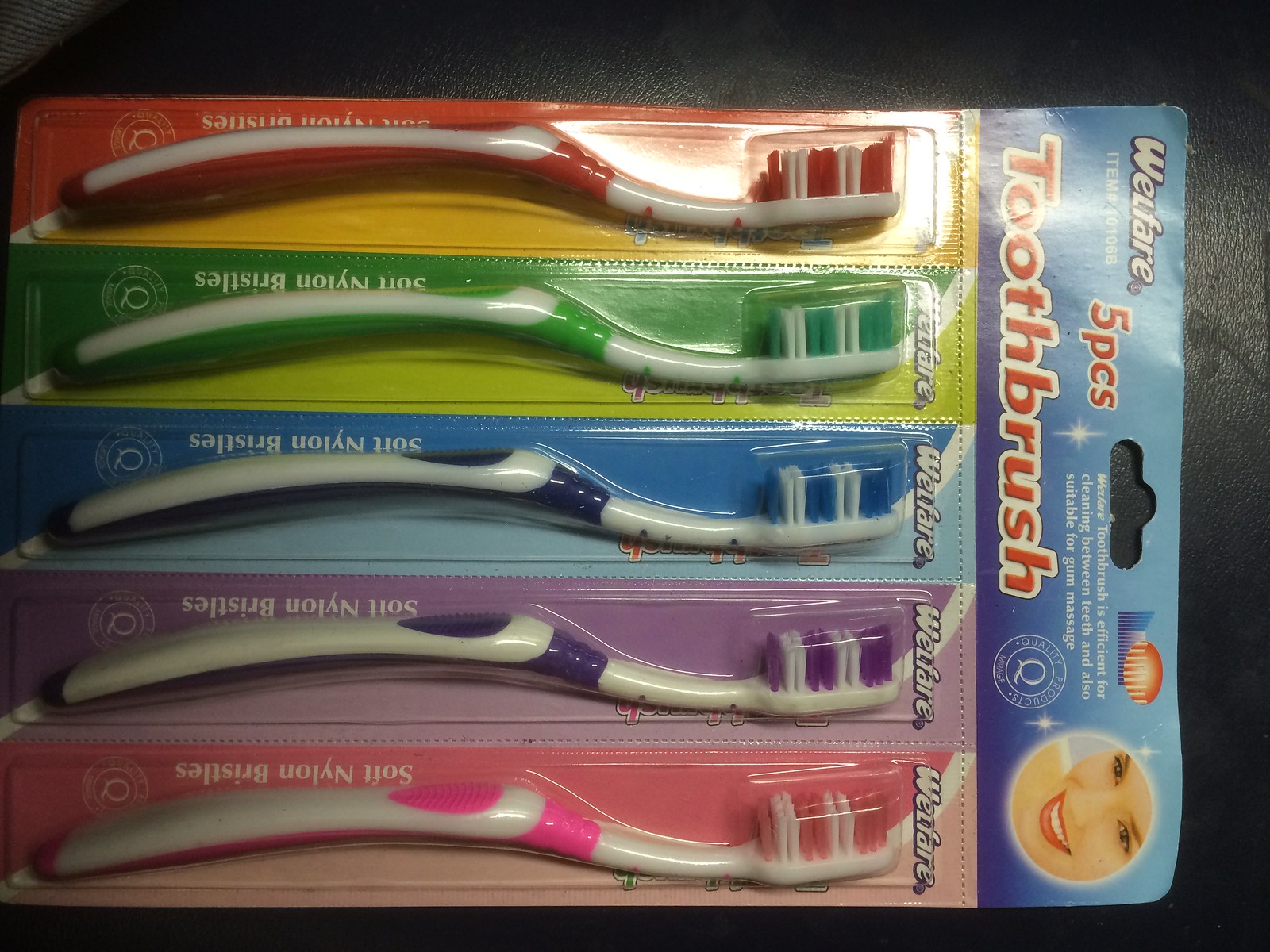This detailed image displays a five-piece toothbrush collection packaged horizontally, with the top oriented to the right and the bottom to the left. The packaging features the brand name "Welfare" in a bubbly text format, shown sideways along the top of each toothbrush. It prominently states "Toothbrush 5 Pieces" in bold red text outlined in white against a gradient background transitioning from light blue to dark blue. The toothbrushes are arranged vertically from bottom to top: red with red and white bristles, green with green and white bristles, blue with blue and white bristles, purple with purple and white bristles, and pink with pink and white bristles—all featuring striped bristle designs. At the bottom right of the packaging, there's a smiling woman's face. Each toothbrush is labeled with "Soft Nylon Bristles" in upside-down text from our view.